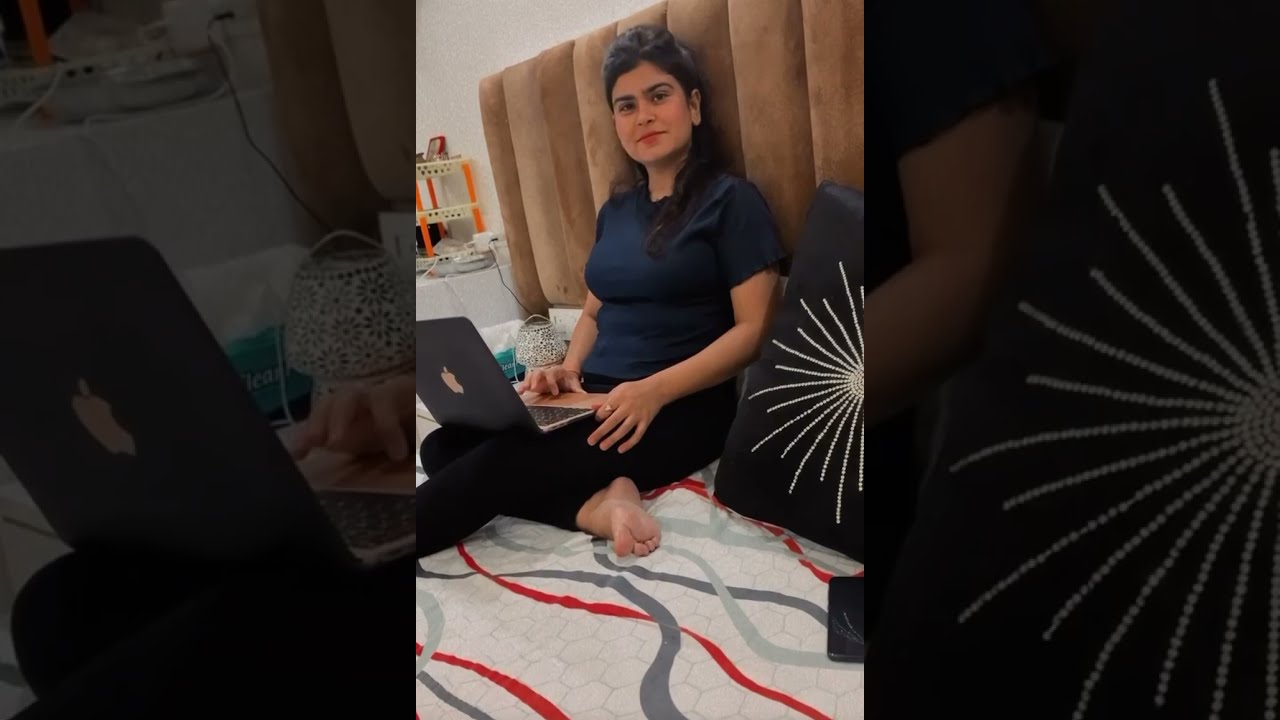In the center of the image, a woman, possibly of Middle Eastern or Indian descent, with olive skin and long black hair is the focal point. Her dark facial features, including dark eyes and red lipstick, complement her attire—a navy blue shirt and black leggings. She is barefoot and seated on a bed, with one leg tucked under the other, engrossed in an Apple laptop perched on her lap. The bed's headboard is cushioned and brown, resembling vertical beams covered in a soft velvet-like fabric.

The bed is adorned with a white sheet featuring wavy red, gray, and silver patterns, adding a playful touch. Beside her, there is a black pillow with a white ornate design reminiscent of a sun or firework. Completing the scene, a bedside table with various items is partially visible. The photo layout includes enlarged, partial segments of the central image on both the left and right sides—highlighting sections of the pillow and laptop, respectively. The woman gazes slightly to her left, seemingly towards the photographer.